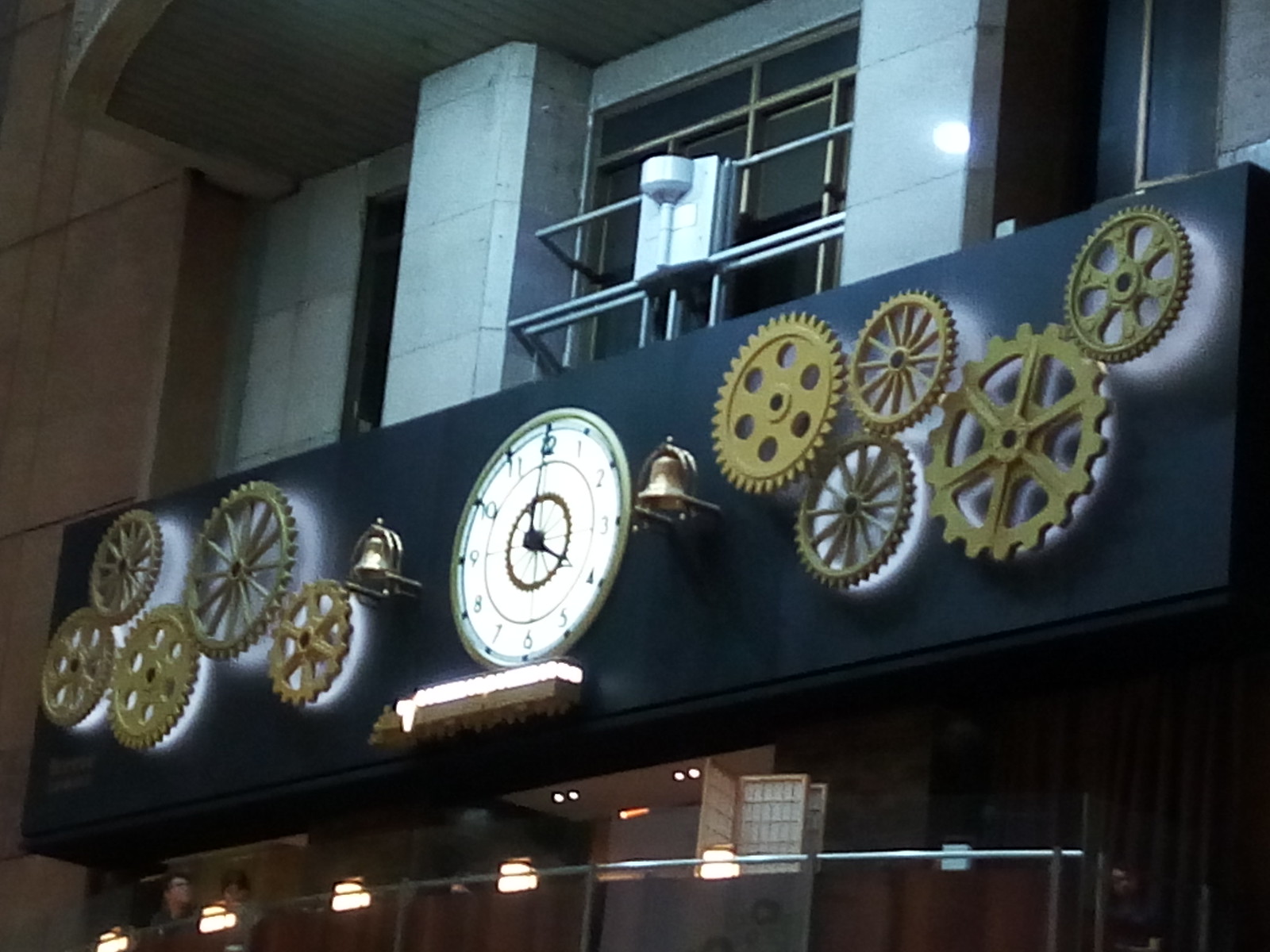The image showcases the intricate blend of interior and exterior elements of a modern architectural structure. Dominating the scene is a striking clock design, featuring a circular white analog clock flanked by two bells, all mounted amidst an array of interconnected golden gears. There are five gears on each side of the clock, varying in size and positioned at different angles, each glowing softly with a bluish illumination, enhancing the mechanical aesthetic.

The structure itself is composed of sleek, silver vertical beams that support a prominent balcony. To the left, the wall juts outward, displaying a rich brown hue that contrasts elegantly with the metallic elements. Below, a pristine white walkway is bordered by glass paneling, ensuring safety while maintaining visual transparency. Two individuals can be seen strolling along this path, adding a sense of scale and life to the scene. Additionally, a blue horizontal strip, running diagonally across the view, adds a pop of color and further depth to the architectural design.